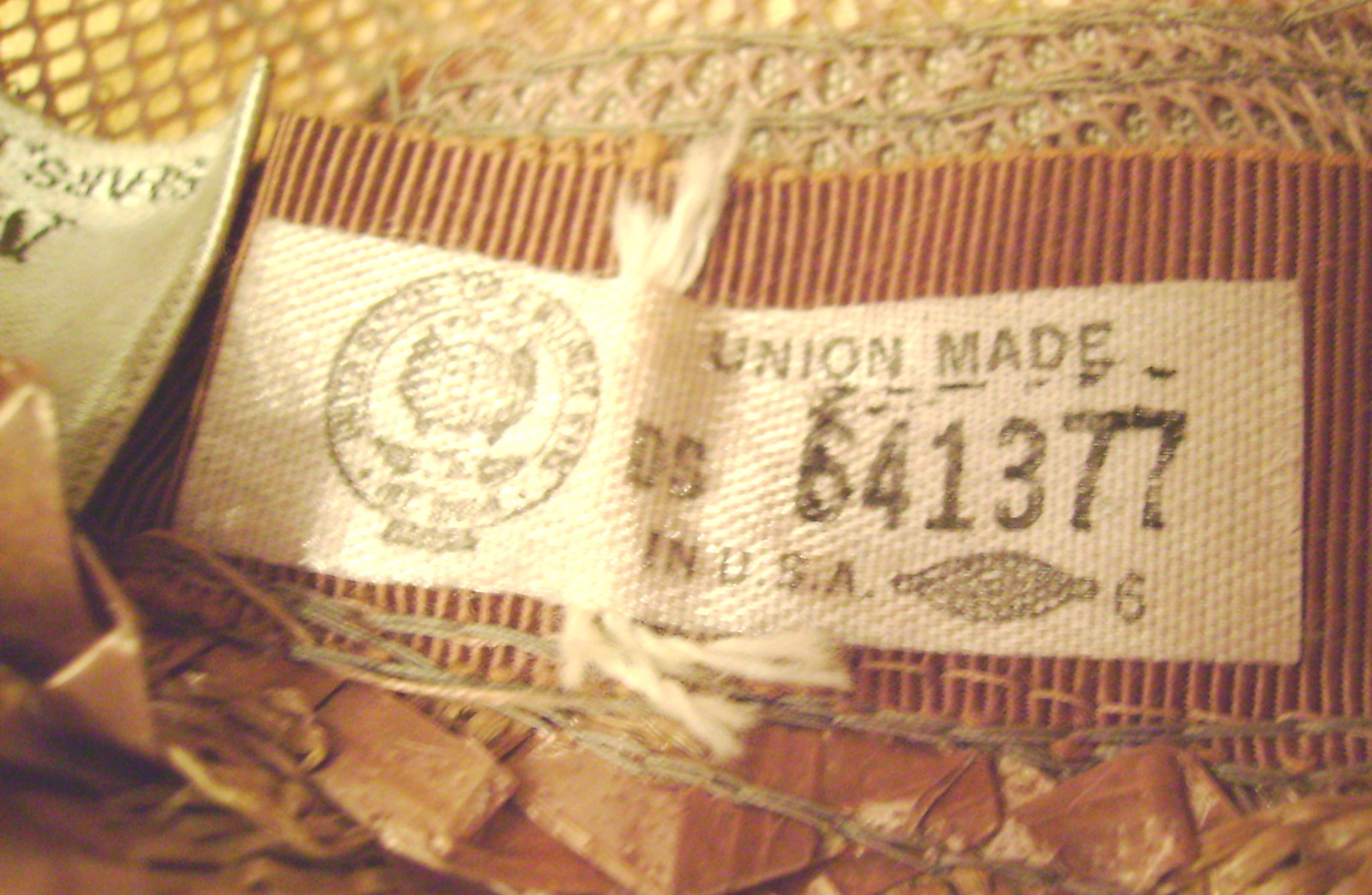This image depicts a close-up of what appears to be a fabric material, possibly crocheted or loosely woven, with two distinct labels attached. The main background fabric is light brown and has the texture of knitted or crocheted material. On the left, there is a metallic label, likely silver or gold, but it's partially obscured and features some text, potentially indicating the size as "Medium," which seems to be embroidered with thread.

The second label, more prominent and placed to the right, has a brown background that resembles wood or carpet. It features a white center with text and symbols. The text on this label includes "Union Made" followed by the code "DS641377" and "Made in U.S.A." This label also includes a small emblem. The overall setting suggests the material could be clothing, fabric, or even a piece of crocheted art, though the exact nature of the item remains unclear due to the intricate and somewhat blurred presentation.